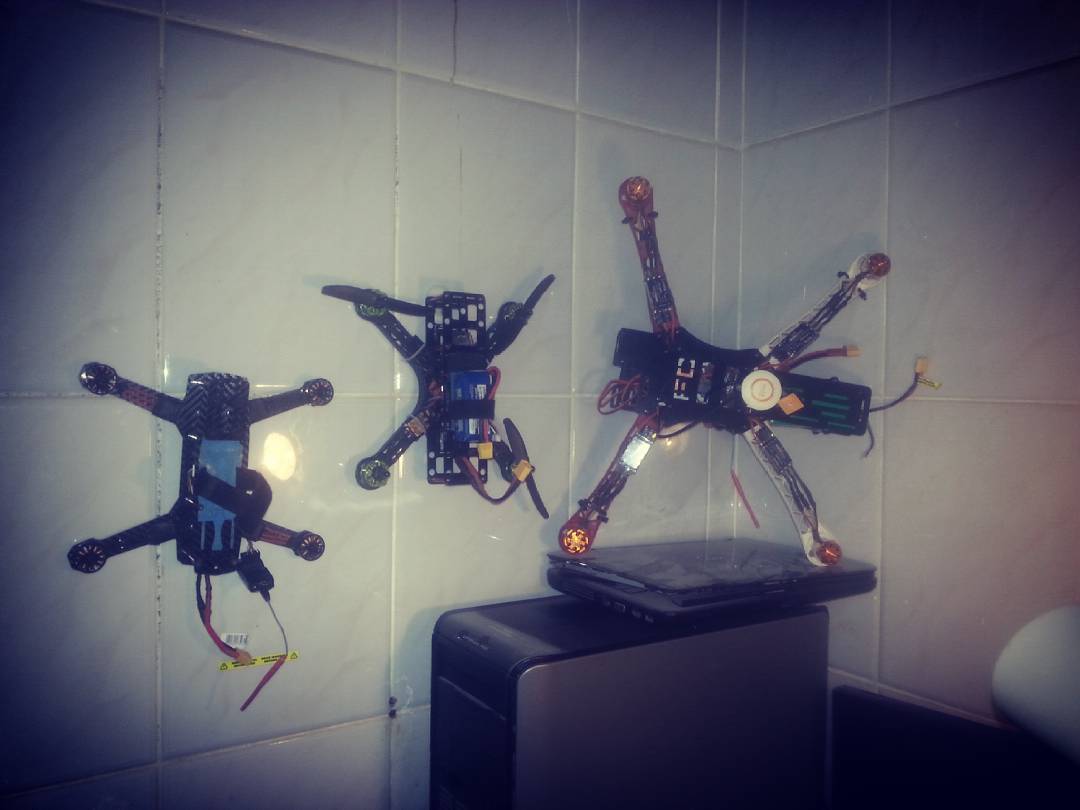In this detailed image, we observe three mechanical devices, likely drones or robots, of varying sizes positioned against a shiny white tiled wall with prominent grout lines. The devices, characterized by their dark bodies, are outfitted with multiple legs that extend outward in an X-formation, with rounded, fan-like structures at the ends of each leg, suggesting they could either float or crawl.

The drones appear to be under construction or in disrepair. The largest drone is leaning against the wall, devoid of any propellers, indicative of ongoing assembly. The second drone appears partially disassembled, missing one or more propellers. The smallest drone is also under some maintenance, intricately displaying its internal components, such as various wires and central rectangular compartments.

At the bottom right of the image, there is a small chair adorned with a white pillow. Mounted atop a black and gray computer tower, there is a laptop computer, which in turn supports one of the smaller drones. The scene is set in a technologically-equipped environment, possibly a workshop or lab, where these mechanical devices are being assembled or repaired.